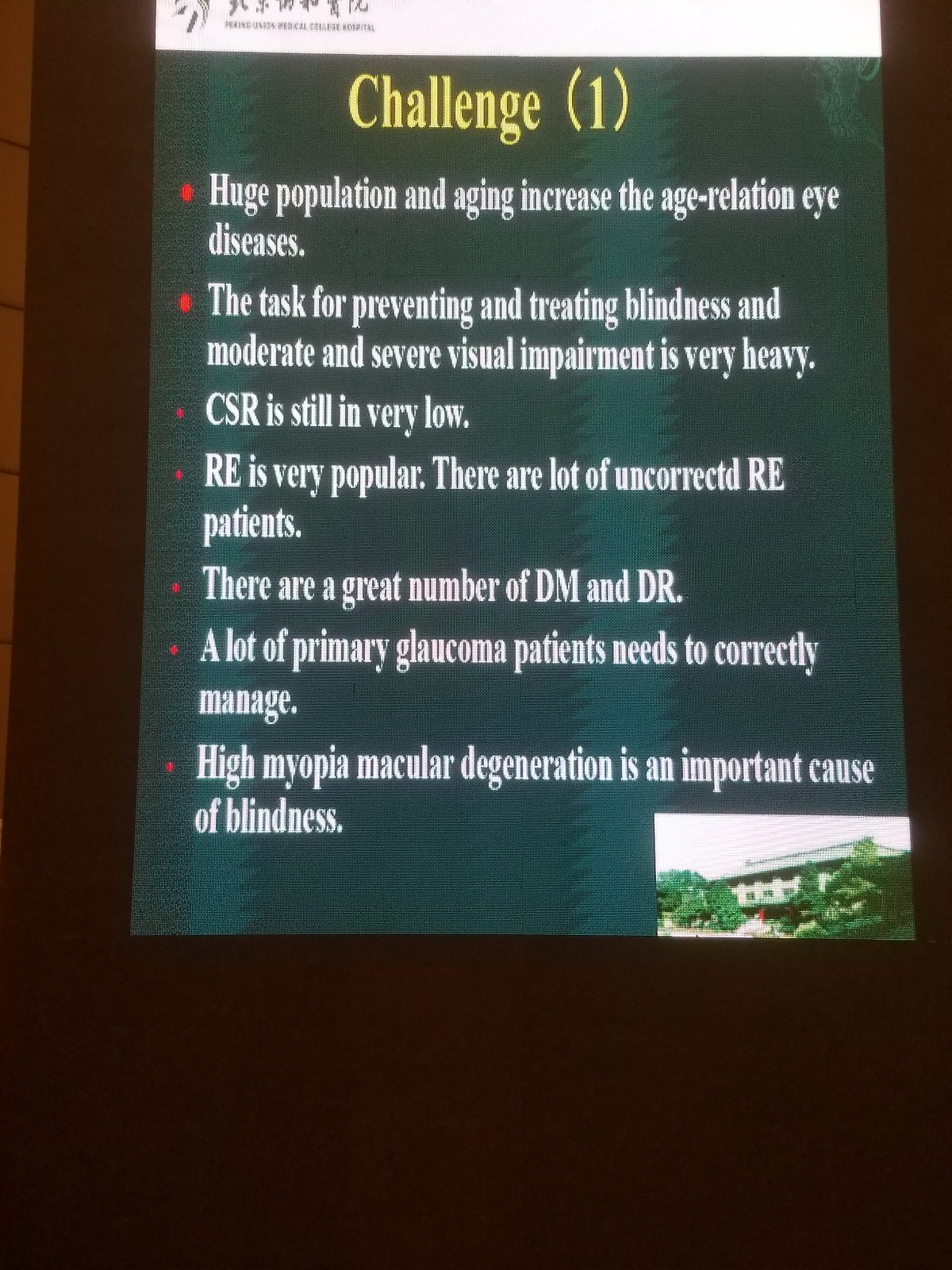This is a detailed color photograph of a green card with a background featuring light green stripes and two light green vertical stripes against a dark green backdrop, giving the appearance of text behind it. The card is placed against a dark red maroon background and includes a white strip at the top with unreadable text in black. Beneath this, in bold yellow letters, the card reads "CHALLENGE 1." Below this heading are several bullet points in red with white text, listing various topics related to eye health: "Huge population and aging increase the age-related eye diseases. The task for preventing and treating blindness and moderate and severe visual impairment is very heavy. CSR is still very low. RE is very popular, with many uncorrected RE patients. There are a significant number of DM and DR cases. A lot of primary glaucoma patients need correct management. High myopia and macular degeneration are important causes of blindness." The lower right-hand side of the image features a picture of a building surrounded by trees, suggesting the location might be an eye health clinic. The sky is visible in the background behind the building.